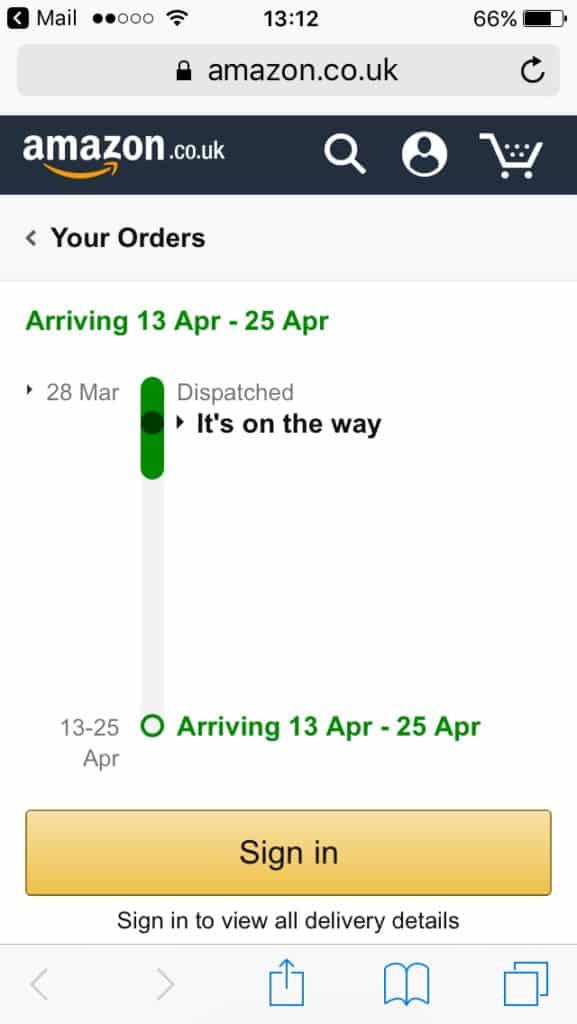The image displays a cell phone screen featuring the delivery status of an Amazon order. At the top of the screen, the text "Mal" appears accompanied by a wireless signal icon and the number "1312." In the upper right corner, the battery level reads "66%." The web address shown is "Amazon.co.uk."

Directly beneath the address bar, the Amazon.co.uk logo appears, followed by icons of a magnifying glass, a person, and a shopping cart. The heading "Your Orders" is prominently displayed. The delivery update states "Arriving 13 April to 25 April" and notes that the package was "Dispatched" on "28 March." A status bar is partially filled in green, showing progress towards the delivery date. The bottom of this vertical bar reiterates the expected arrival between "13 to 25 April."

Below this, a yellow rectangle with the text "Sign In" asks the user to sign in to view all delivery details. At the very bottom of the screen, navigation icons include a left arrow, a right arrow, an upward arrow in a box, an open book, and two overlapping squares.